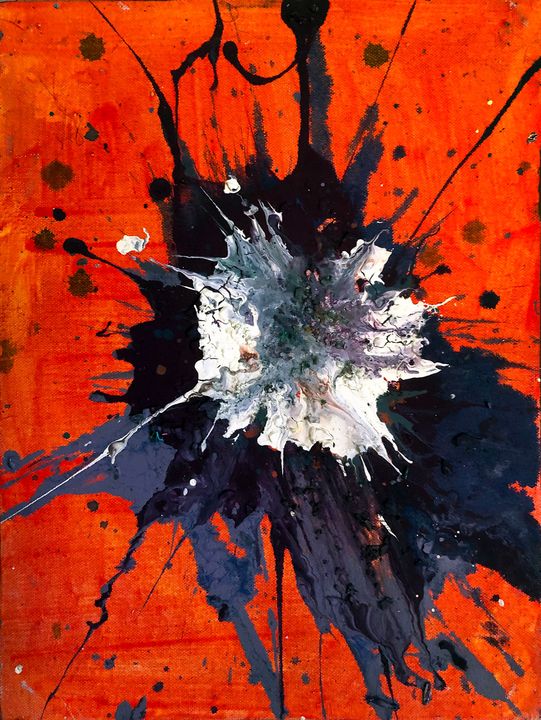This image is a rectangular abstract painting on a canvas that extends vertically from top to bottom. The backdrop of the painting features a rich red color interspersed with various streaks and brushstrokes of red and orange hues, providing a textured foundation. Layered atop this vibrant background is a prominent gray splatter mark, which stretches across the canvas and appears to drip down in places. Positioned centrally over the gray is a bold black splatter, sending dots and streaks that reach toward the bottom left, top right, and beyond. Overlaying these layers is a white splatter mark, more concentrated in the center and supplemented with hints of gray and purple. This final white layer also emits smaller splatters, adding to the complexity and depth of the painting. The composition is a dynamic interplay of colors and textures, devoid of any textual or figurative elements, embodying pure abstract expression.